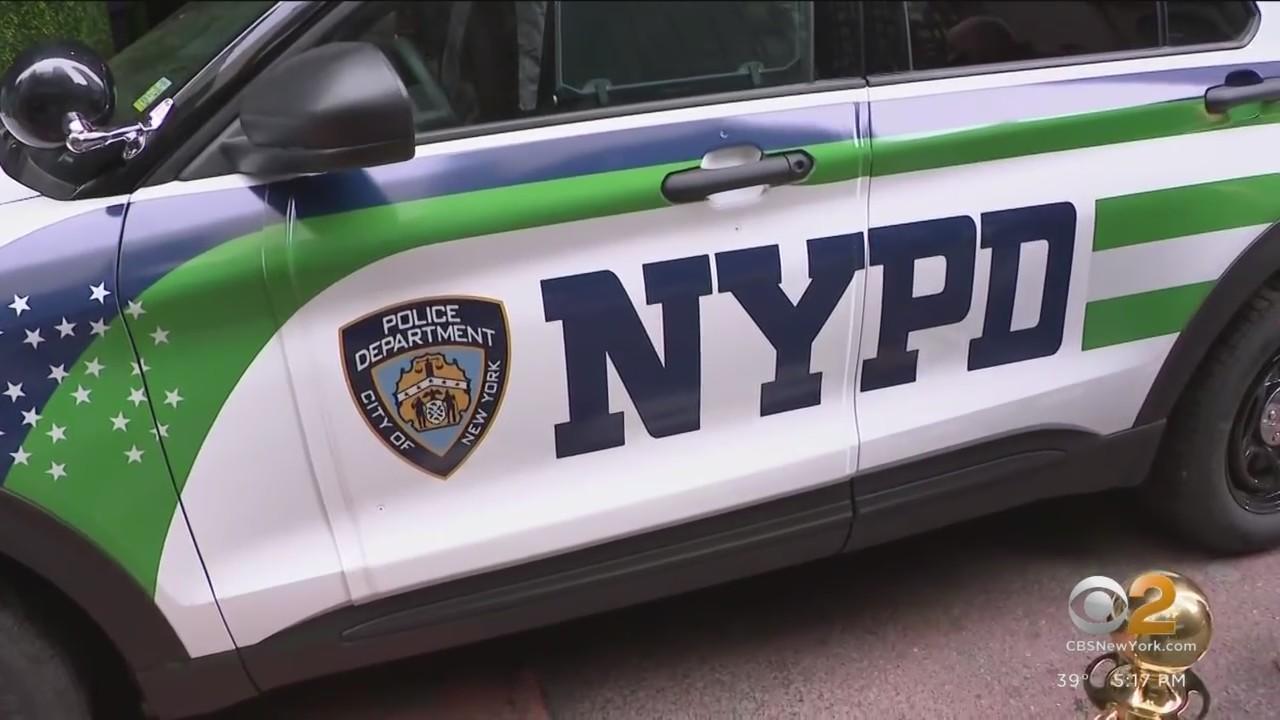Screenshot from a CBS New York newscast shows a close-up of a NYPD police car. In the bottom right corner, the CBS logo, marked with a silver "I" and the number "2" for Channel 2, is visible along with the text "cbsnewyork.com." The display also indicates that the temperature is 39 degrees and the time is 5:17 PM, though the white text is somewhat challenging to read against the background.

Dominating the image is the white police car, featuring distinct green and blue stripes, and an additional green and white stripe above the rear wheel. The close-up focuses on the driver’s side, which displays the official logo of the "Police Department, City of New York" in a badge shape on the driver’s door. The acronym "NYPD," rendered in navy blue, spans between the driver’s door and the rear passenger door, with "NY" on the former and "PD" on the latter. A small portion of the road is visible in the bottom right corner of the image, providing context to the scene.